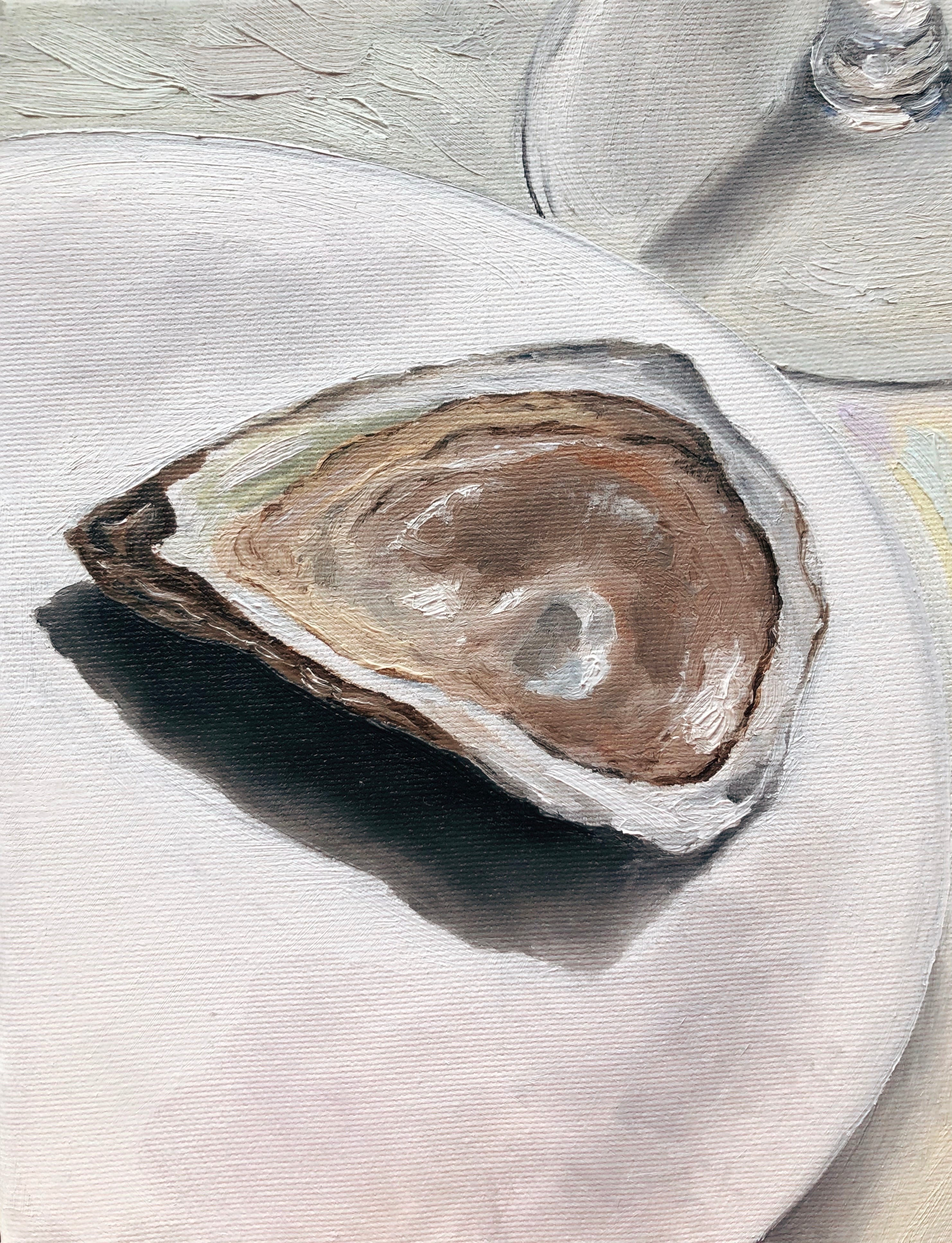The image is a detailed oil painting showcasing a close-up view of what appears to be an oyster shell, depicted with intricate textures and colors. The half-shell rests on a stark white plate, with a detailed rim of dark brown. The interior of the shell displays a mixture of brown and red tones, with a notable white area in the center. This plate sits on a surface that resembles a multicolored gray tablecloth or wooden table, evidenced by textured and shaded brushstrokes. In the upper right-hand corner, part of a glass object—possibly a vase or candlestick—is subtly visible, introducing pale yellow and light blue hues, alongside a faint pink and purple paintbrush handle. The overall composition focuses on the central oyster shell, presenting it with a rich, almost edible realism, while the surrounding elements add depth and an artistic layered aesthetic.